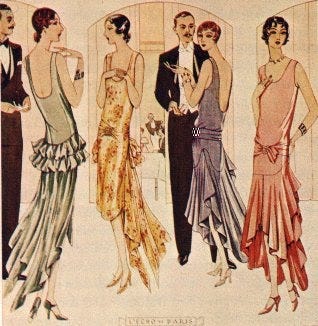This vibrant painting depicts a sophisticated 1920s party scene with elegantly dressed men and women. On the left, a man in a black tuxedo, partially cut off by the frame, stands near a fair-skinned woman in a green, drop-waisted slip dress with a streamlined tulle bottom. To her right, another woman, adorned in a yellow slip dress, shares the same era-defining fashion with sleek, tightly styled dark hair and accessories such as bracelets and necklaces.

A man with a mustache and dark hair, also in a black tuxedo but with a white tie, engages in conversation with a light brown-haired woman dressed in a long, purple drop-waisted gown. On the far right, a woman stands gracefully in a pinkish-red dress with a similar drop-waist design, sporting dark hair and high heels.

The background reveals an arched opening draped with a curtain, through which a table set for diners is visible. A waiter appears to be serving the seated guests. The composition captures the essence of the Roaring Twenties, complete with the iconic flapper fashion, characterized by their short wavy hair, frills, bows, and jewels on their dresses. The bottom of the artwork hints at a Parisian locale, adding to the scene's allure and sophistication.